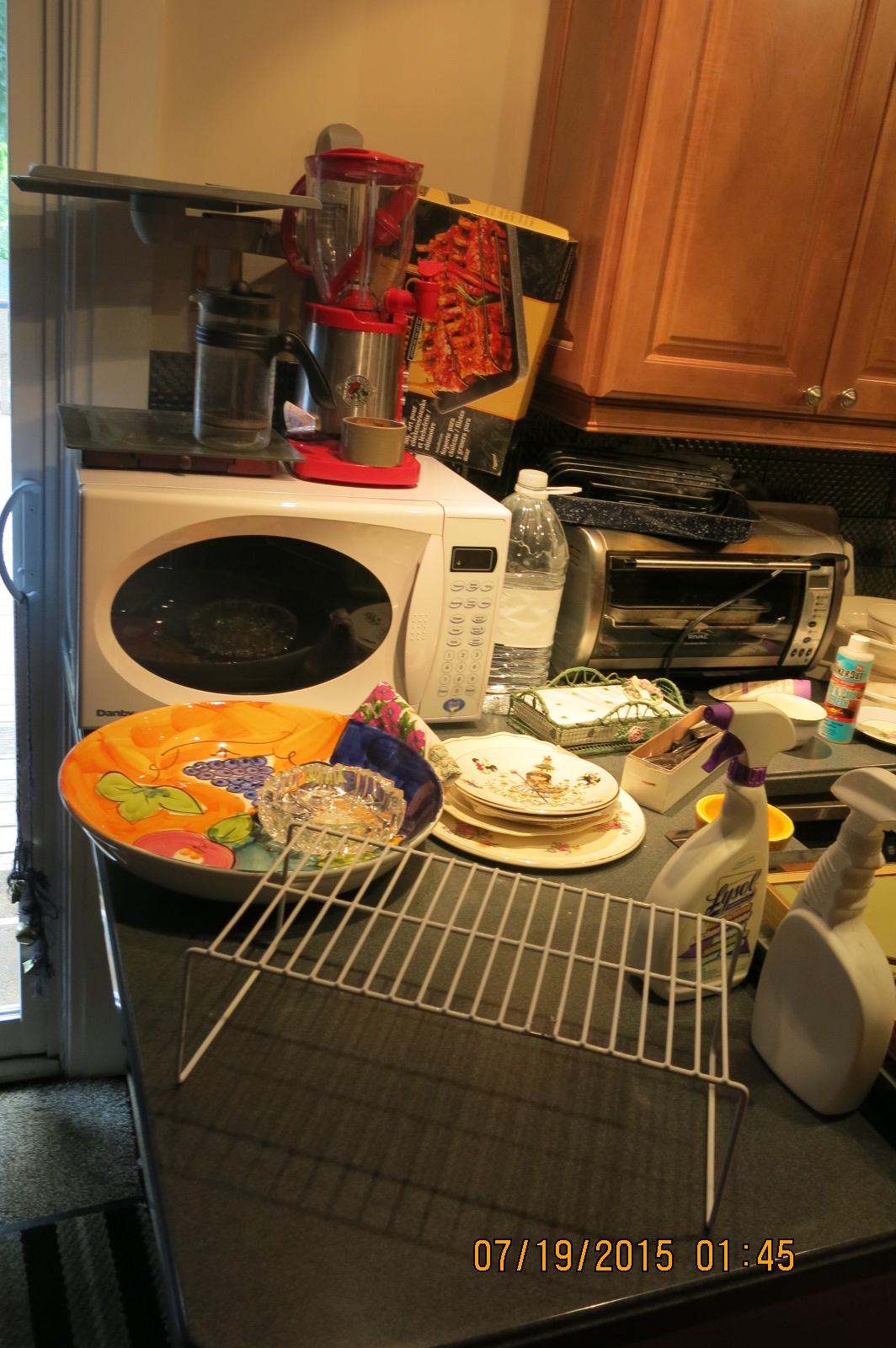This photograph captures a kitchen counter cluttered with various items. Dominating the scene are five dirty dishes scattered across the black countertops, alongside an ashtray. To the left, a white microwave with red and black containers perched on top is visible. Beneath the microwave sits a white dish rack flanked by two spray bottles, one of which is a Lysol cleaner. The upper right corner reveals a brown cabinet door. To the far left, a door with a glass panel and a brown rug are seen. On the right side, a gray toaster oven is present, accompanied by a water bottle. Adjacent to the toaster oven, more dishes are piled up, though they extend out of the frame. A blue and red smaller bottle, a green napkin holder with white napkins, a small box of utensils, and a yellow bowl are also noticeable, adding to the array of items on the counter.